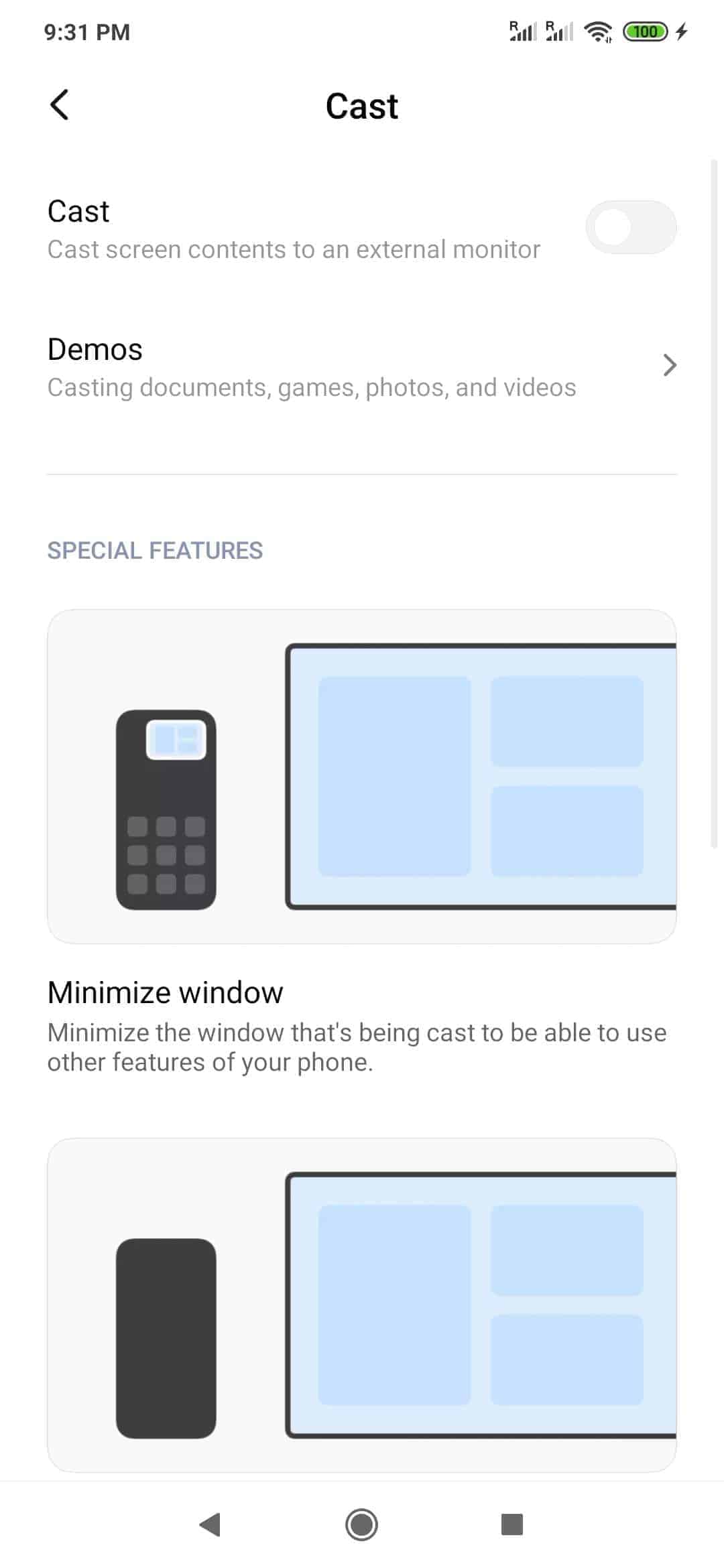The image is a screenshot set against a pristine white background. In the upper left corner, the time is displayed as 9:31 PM. The upper right corner features a black icon indicating a Wi-Fi connection and a fully charged battery at 100%. Centrally positioned, bold black text reads "CAST" with an arrow pointing to the left. Directly beneath, the word "CAST" appears again in smaller black text. Further down, in gray text, it states, "CAST screen contents to an external monitor." 

Following this, the text reads, "Demos, casting documents, games, photos, and videos," with a right-facing arrow beside it. Below this section, in gray text on a white background, are the words "Special features." On the right side and slightly below, there is a blue rectangle outlined in black, labeled "Minimize window." The accompanying text reads, "Minimize the window that's being cast to be able to use other features of your phone." An illustration beneath this shows a black cell phone with a blue box in the upper right corner.